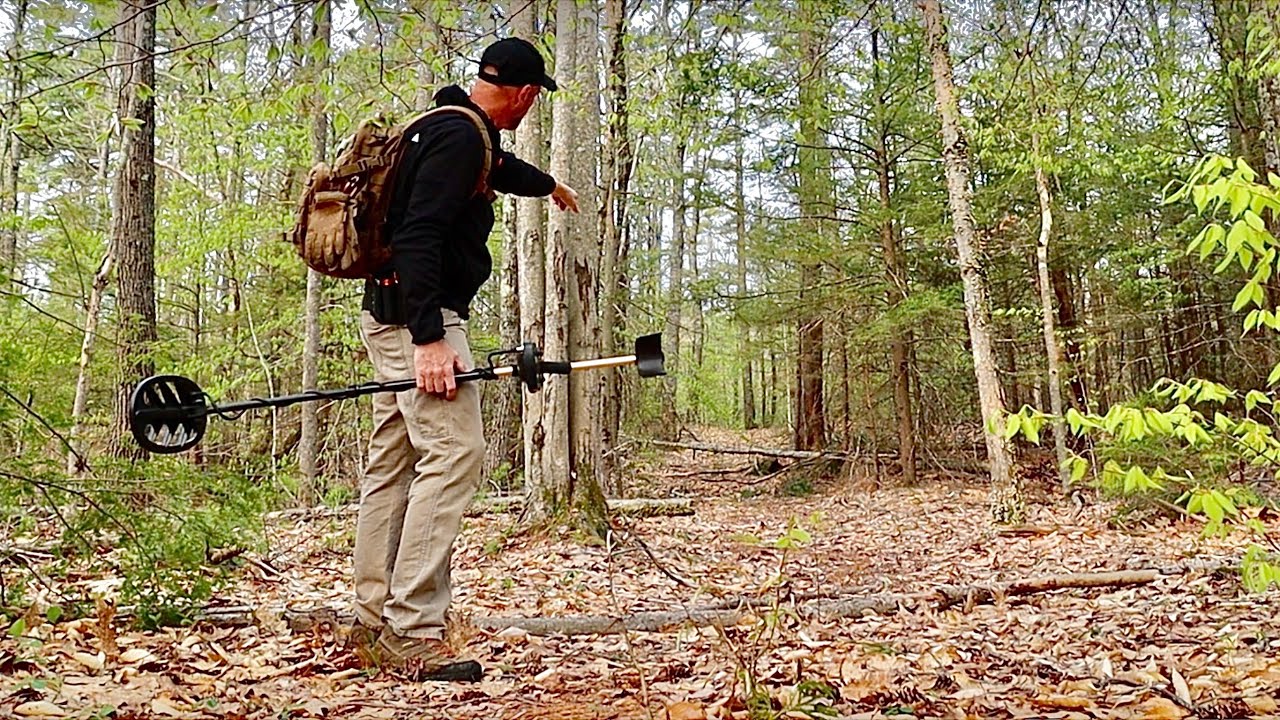In this detailed outdoor scene set in a dense forest, the gray sky peeks through a canopy of varied green and leafless tree branches, creating a contrast that defines the early spring setting. The forest floor is a tapestry of dead brown leaves, broken branches, and chipped wood, partially covering a discernible pathway. The pathway meanders through a mix of tall deciduous trees and some conifers, some of which have begun to show new foliage.

Standing just off-center to the left is a man, viewed from his right profile, dressed warmly for the outdoors. He sports brown hiking boots with black soles, khaki pants, and a black long-sleeve jacket with a hood. A black baseball cap shades his face. His brown backpack is snugly secured on his back. In his right hand, he firmly grips a long pole, specifically a metal detector with a distinctive round black piece at the bottom, marked by several holes and black lines. This device features a partly white shaft with two black components.

His left arm is extended, index finger pointing purposefully down the trail, possibly towards a fallen tree that lies across the path, implicating either a discovery or a direction of interest. The entire scene captures a moment of exploration and intrigue in a secluded part of nature.